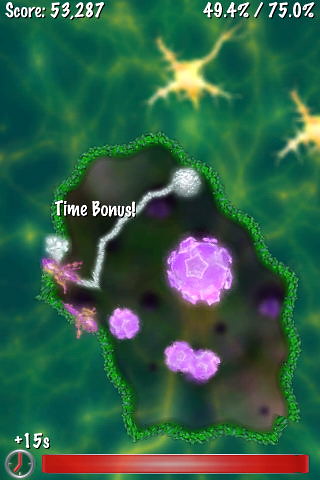The image appears to be a screenshot from a puzzle game, likely designed for mobile devices. The upper left corner displays a score of 53,287 in white lettering, indicating the player's current points. On the right side, there are percentages—49.4% and 75%—possibly representing progress or completion rates.

The central area features a green-hued environment, resembling a pond, surrounded by a green trim. This area is dotted with glowing purple lilies, enhancing the mystical ambiance. Within the pond, a creature that resembles either a frog or a spider is seen swimming, adding a dynamic element to the scene. Above the creature, the words "Time Bonus" are displayed, hinting at a timed challenge or reward.

A grayish-white streak traverses the pond, perhaps indicating the path taken by the creature or an area of interaction. At the bottom of the image, there is a timer reading "+15 S" next to a red bar, suggesting a countdown or an additional time bonus. Overall, the vivid colors and various game elements imply that this screenshot is indeed from an engaging and colorful mobile puzzle game.